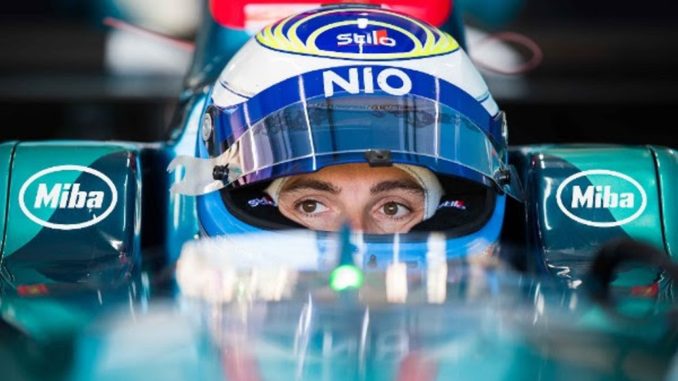This close-up photograph captures a race car driver seated in his vehicle. The image focuses on the man, whose dark brown eyes and eyebrows are prominent as he looks to his right with a serious expression. He is wearing a large helmet, predominantly blue with white accents, and a detailed design featuring a bright blue bottom, a dark blue stripe, and blue circles surrounded by yellow at the top. The helmet's visor is raised, revealing more of his face from about the mouth upwards. The helmet displays the words "NIO" across the front and "STILO" on top in white lettering. Behind him, part of his car is visible, showcasing a light green and dark blue color scheme with a logo reading "M-I-B-A" in a white oval. The bottom quarter of the photograph is out of focus, adding a blurred effect.